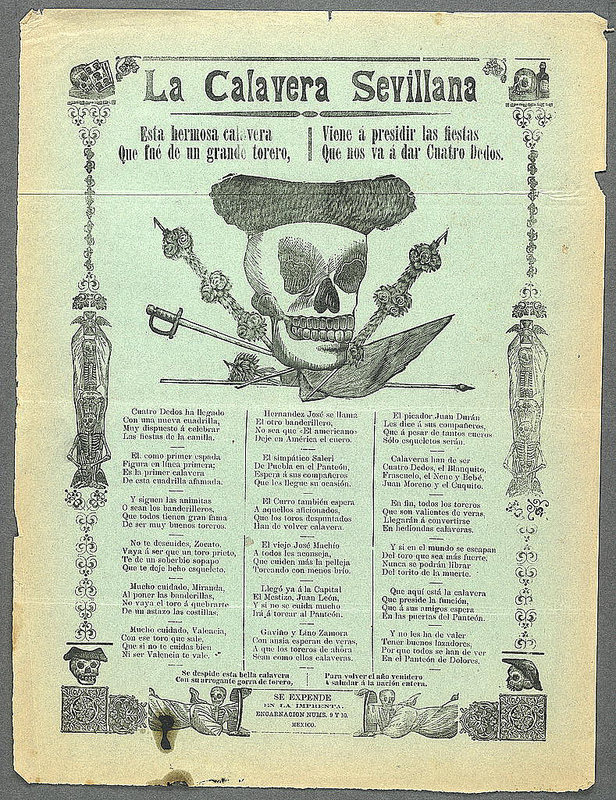The image resembles an old Spanish newspaper, pamphlet, or poster, titled "La Calavera Sevillana." It features a central emblem of a skull, adorned with a hat reminiscent of a bullfighter's, flanked by crossed swords and possibly a paintbrush or flag. The text, primarily in Spanish, is arranged in three vertical columns beneath a bold headline. The background is cream-colored with black text, and there's a subtle blue hue at the center. The borders are intricately decorated with images such as skulls, jewelry, angels holding a banner, and possibly wine bottles, reflecting an 18th or 17th-century Spanish style.